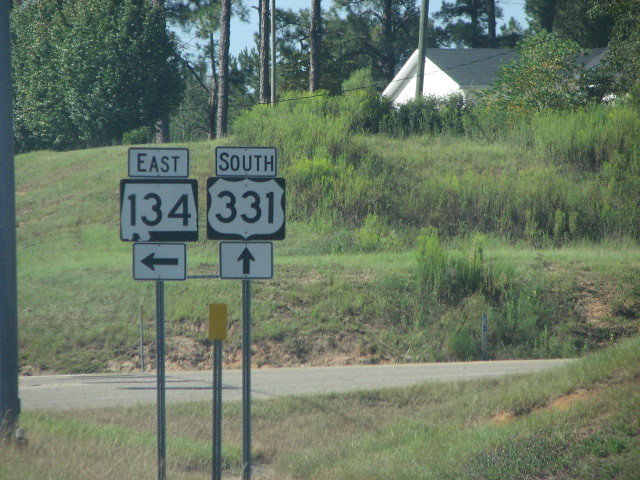This detailed photograph captures a scenic roadside view dominated by two highway signs mounted on grey metal poles. The left sign indicates "East 134" with a left-pointing arrow, while the right sign denotes "South 331" with an upward-pointing arrow. Each sign features a white rectangle background with black text and arrows. In the foreground, the signs are positioned on a grey stone pavement next to a grass verge. The landscape extends to a grassy field leading up to well-kept, mown hills interspersed with patches of longer vegetation. A row of bushes stretches across the middle of the scene, with an apple tree just visible peeking over them. Beyond the bushes, the roof and white siding of a house are partially seen, with its gray roofing felt contrasting against the foliage. Tall trees with slender trunks rise in the backdrop, adding depth to the composition. A telephone pole with visible wiring stands in front of the house, further punctuating this picturesque view.